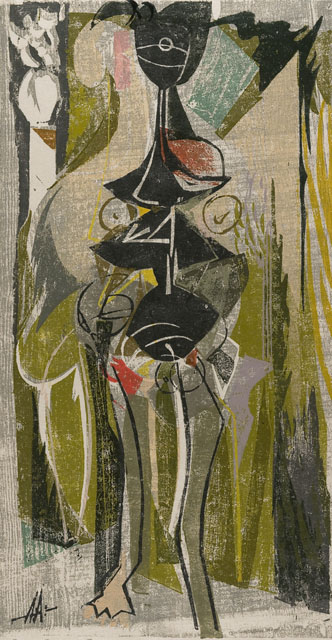This vibrant and abstract painting features what appears to be a humanoid figure situated at the center, crafted with a rich palette primarily comprising black, olive green, and dark green, accented with sporadic touches of red. The figure's legs, light green with duck-like fins at their ends, emanate a surreal, non-human quality. The midsection of the form is irregular in shape, predominantly black, and intriguingly marked with stacked triangular forms that transition into a rounded base where the legs begin. The torso seems fragmented and intersects with the head-like element, which lacks definitive facial features but is characterized by black color with white lines and two black wavy strands that may signify hair. Around the chest area, there's a notable red structure contributing to the figure's strange anatomy.

In the background, the use of turquoise, green, gray, cream, and light blue hues enriches the painting with a sense of depth and chaotic harmony. Circles and other irregular shapes punctuate the abstract landscape. Notably, there are two letters 'A' inscribed at the bottom left corner, serving as the painter's signature. Despite the detailed rendering, the piece remains elusive, teetering between the resemblance of a person and a series of abstract forms, suggesting movement towards the observer or presence within a defined space.